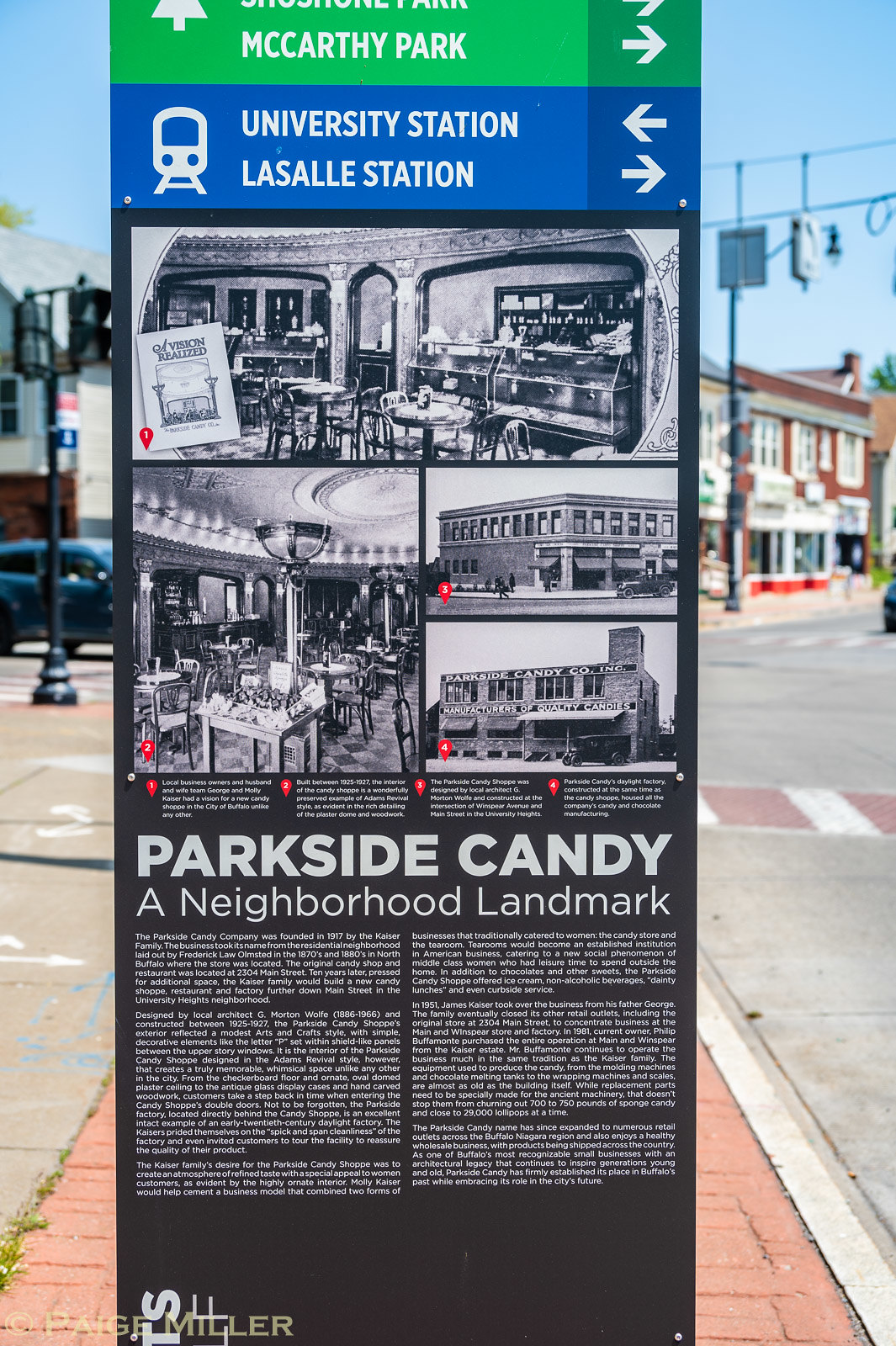This color photograph, captured in portrait orientation, showcases a vertical neighborhood landmark sign positioned on a red brick sidewalk in an urban setting. The sidewalk is on the left, and a paved street is visible on the right, flanked by commercial buildings configured in a strip, partly visible in the background. The sign, constructed of what seems to be a sturdy material like cardboard, is topped with directional signage. The green signage on top reads "McCarthy Park" and features an arrow pointing to the right and straight ahead. Below this is a blue strip indicating "University Station, LaSalle Station" with a white bus icon and arrows pointing in both directions.

The sign prominently displays four vintage black-and-white photographs that offer glimpses into the neighborhood's historical landscape. The top photograph depicts a restaurant scene, followed by an interior shot of a restaurant setup below it. Adjacent to these are two photographs of buildings, one of which prominently features "Parkside Candy Co., Manufacturer of Quality Candies." Beneath the images, in bold white text, is the label "Parkside Candy," followed by the subtitle "A Neighborhood Landmark." Although partly obscured, more detailed descriptions seem to be provided in smaller white text towards the bottom, set against a black background. The photographic style is a detailed representationalism realism, capturing and commemorating the rich local heritage of the area.